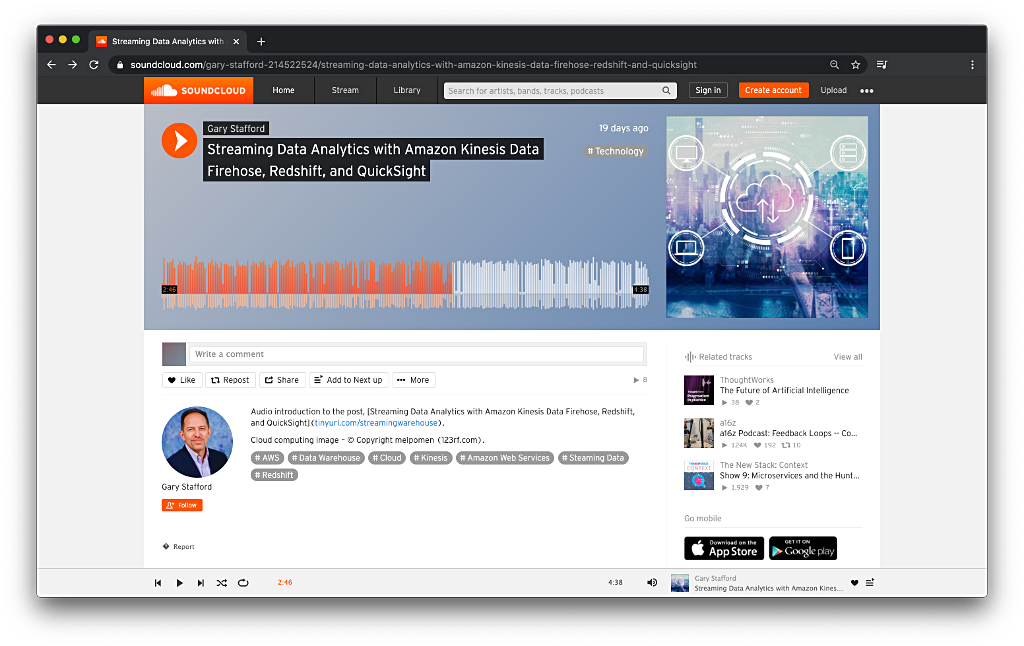This is a detailed screenshot of the SoundCloud website. The address bar at the top left confirms the site as SoundCloud.com. The characteristic layout and color scheme—orange, white, blue, and purple—identify it unmistakably. 

At the top of the page, the SoundCloud navigation bar is prominently displayed. The SoundCloud logo, situated on the far left, features an orange background with a half-cloud design. The left side of the cloud morphs into a series of lines resembling sound waves, symbolizing the transformation of sound into a cloud. 

Adjacent to the logo are several navigation options: Home, Stream, and Library tabs, followed by a search bar. Further along, there are Sign In and Create Account buttons—the latter is orange for emphasis—and an Upload button. A three-dot icon at the end of the bar offers more options when clicked.

The main content visible on the screen indicates that the user is exploring a track by Gary Strafford titled "Streaming Data Analytics with Amazon Kinesis Data, Firehose, Redshift, and QuickSight," capturing the essence of the user's current engagement with detailed SoundCloud offerings.